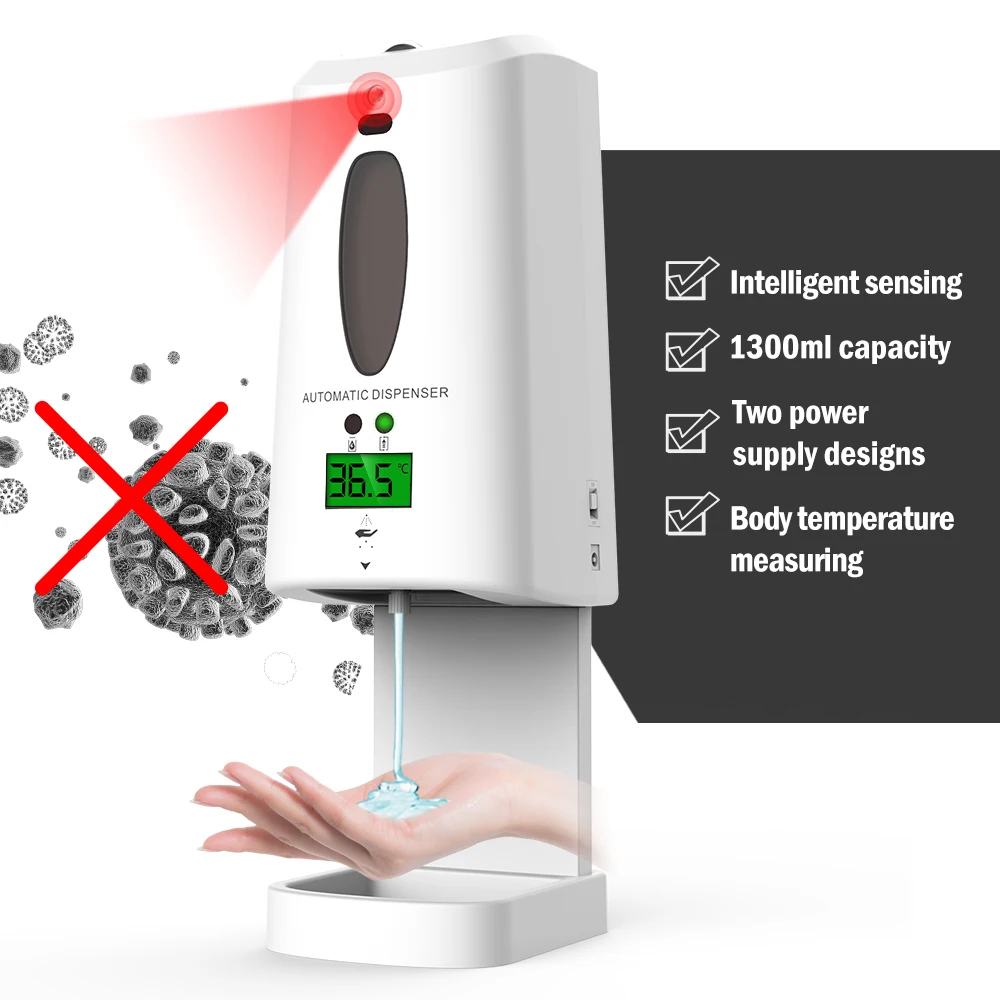The image showcases an advertisement for a white automatic soap dispenser, set against a plain white background. The soap dispenser is attached to a singular vertical wall and faces slightly to the left, with its right side closer to the viewer. A small red light at the top indicates the sensor radius. Below this, there's an oval window showing the soap level inside. Beneath the window, the words "automatic dispenser" are displayed, followed by two indicator circles, one green and currently lit, and one black. Below these circles is a green digital display reading "36.5C".

At the base of the dispenser, soap is being dispensed onto a hand, with a small tray beneath to catch any excess soap. To the left of the image, a red X marks over illustrations of germs, emphasizing hygiene. On the right side, a black label with four check-marked boxes highlights the features: "intelligent sensing," "1300 mL capacity," "two power supply designs," and "body temperature measuring."